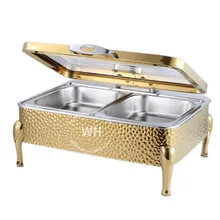This image features a detailed, elegant lunch catering tray, primarily used for formal events such as outdoor gatherings or weddings. The rectangular tray, which has a sophisticated gold exterior that appears to be hand-pounded, stands on four gold legs. The lid, propped open and hinged, is distinct with its gold trim and a center section that is either see-through or made of stainless steel. Adding to its opulence, the handle on the lid is made of chrome metal. Inside the tray are two separate stainless steel holding pans, perfect for serving different entrees or sides such as mashed potatoes. The front of the tray features a circular watermark with the capital letters "W" and "H" emblazoned in its center. The tray is angled slightly to the right, with the lid showcasing an additional stainless steel surface. The photo has a predominantly white background, which accentuates the gold and silver tones of the catering tray, making it the centerpiece of the image.